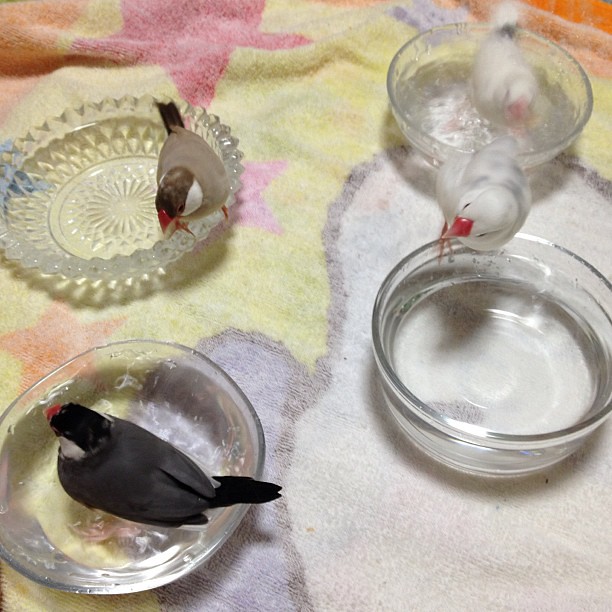The image depicts four clear glass bowls of various designs and textures, arranged on a colorful tablecloth featuring a puzzle-like pattern with yellows, blues, whites, and pink-colored stars. The bowls are skewed slightly from the lower left to the upper right. The bowl at the back left is flatter with curved sides and etched designs, while the one in the left foreground is round with curvy edges. The right-front bowl is taller with two rims and ridges, whereas the back-right bowl is shallower with a frosted texture. Each bowl appears to be filled with water and contains small birds. The front-left bowl hosts a darker-colored bird with a black crown, back, and tail feathers, and a red beak. Behind it, the back-left bowl contains a tan-colored bird with a black head and white cheeks. The front-right bowl holds a white bird with an orange beak, and behind the back-right bowl, another light-colored bird, white with light gray feathers, is either in or near the bowl. The photograph is taken from above, capturing the clear glass containers and their small avian occupants on the vibrant, star-patterned tablecloth.